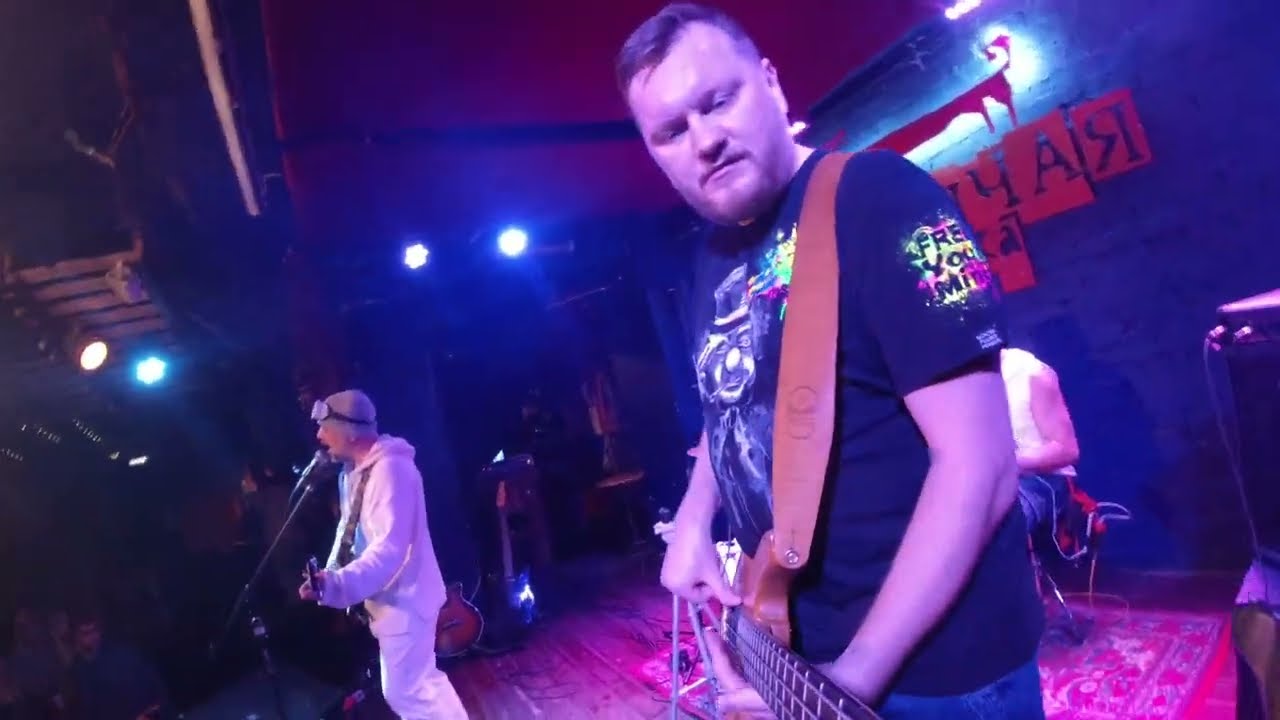In this image, a live music performance is captured with detailed emphasis on the musicians and the stage setup. In the foreground, a bass player is seen wearing a black T-shirt, blue jeans, and a brown strap around his brown wood-colored bass guitar. He has short hair and is looking almost directly at the camera. To his left, a singer is dressed in a full white outfit, including a hoodie and pants, with a pair of goggles around his forehead. He is holding a guitar and appears to be singing into a microphone. Behind the bass player, the partial figure of a drummer is visible, identifiable only by his left arm. The stage floor is covered with a Persian-style rug featuring a Paisley design, and a barely discernible red logo is set against a black backdrop. The stage and its surroundings are bathed in a purplish hue from the lighting, and on the right-hand side of the image, part of a bongo-style drum can be seen.